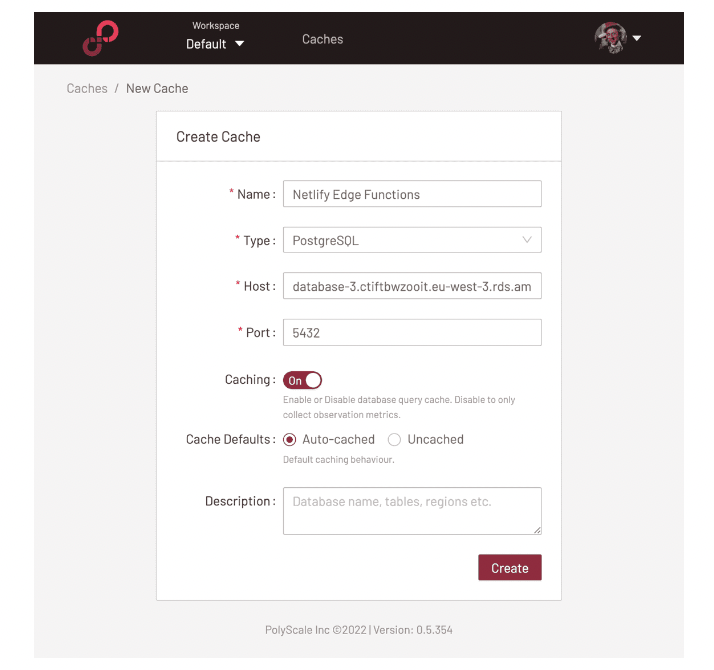In the top right corner of the image, there is a profile picture featuring an image of Willy Wonka with his hand on his chin. Adjacent to the profile picture, there is a white drop-down arrow. In the top middle section, the word "Cassius" is displayed, with the term "workspace, default" to its left. Next to "default," another drop-down arrow is visible. On the top left of the image, there is a logo resembling a red, diagonal infinity symbol pointing towards the top right.

Centrally located in the image, there is a rectangular dialog box titled "Create Cache" at its top left corner. This box contains several labeled fields arranged vertically for entering text. From top to bottom, the fields are labeled: "Name," "Type," "Host," "Port," "Caching," "Cache Default," and "Description." Next to the "Caching" field, there is an on/off toggle button. The "Description" field features the largest text input area, represented by a thick rectangle.